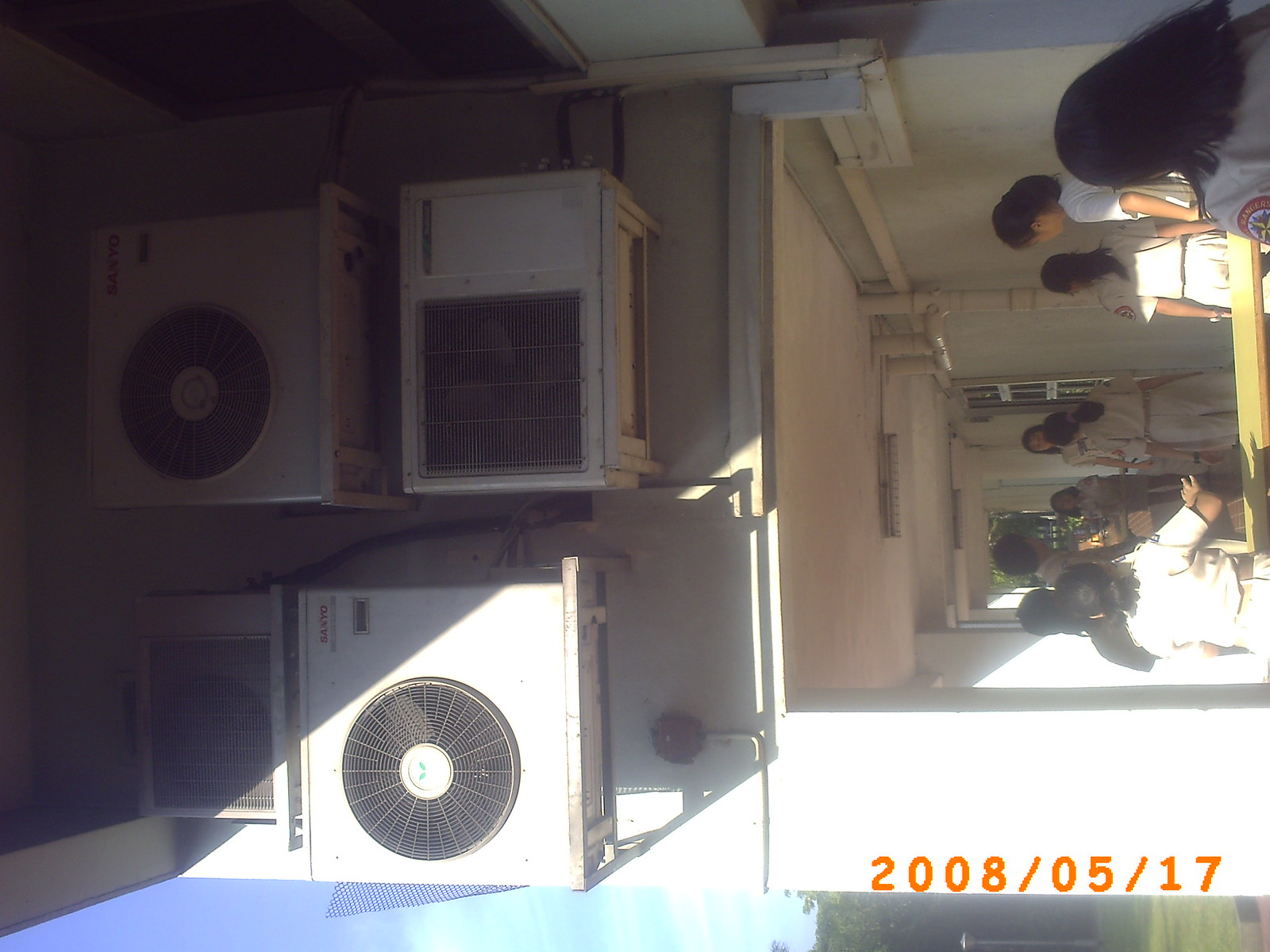This photograph, dated 2008-05-17, captures a group of predominantly Asian individuals, mostly females and possibly one male, gathered outside a building. The image is tilted 45 degrees to the left and appears to be taken from the perspective of someone standing close to the structure. The group is positioned in a hallway-like corridor beneath some pillars, by white walls. They all have dark hair and are wearing what look like uniforms, similar to those worn by Girl Scouts or Boy Scouts, mostly beige in color. Notably, there are four prominent air conditioning units mounted on the building, with various designs: two traditional circular fans, and two with different shapes, one covered by a square grid. Above the wall, there's also a visible fire alarm. The sunlight is evident in the scene, casting light on the group as they stand and interact, possibly engaged in a tour or activity of some sort.